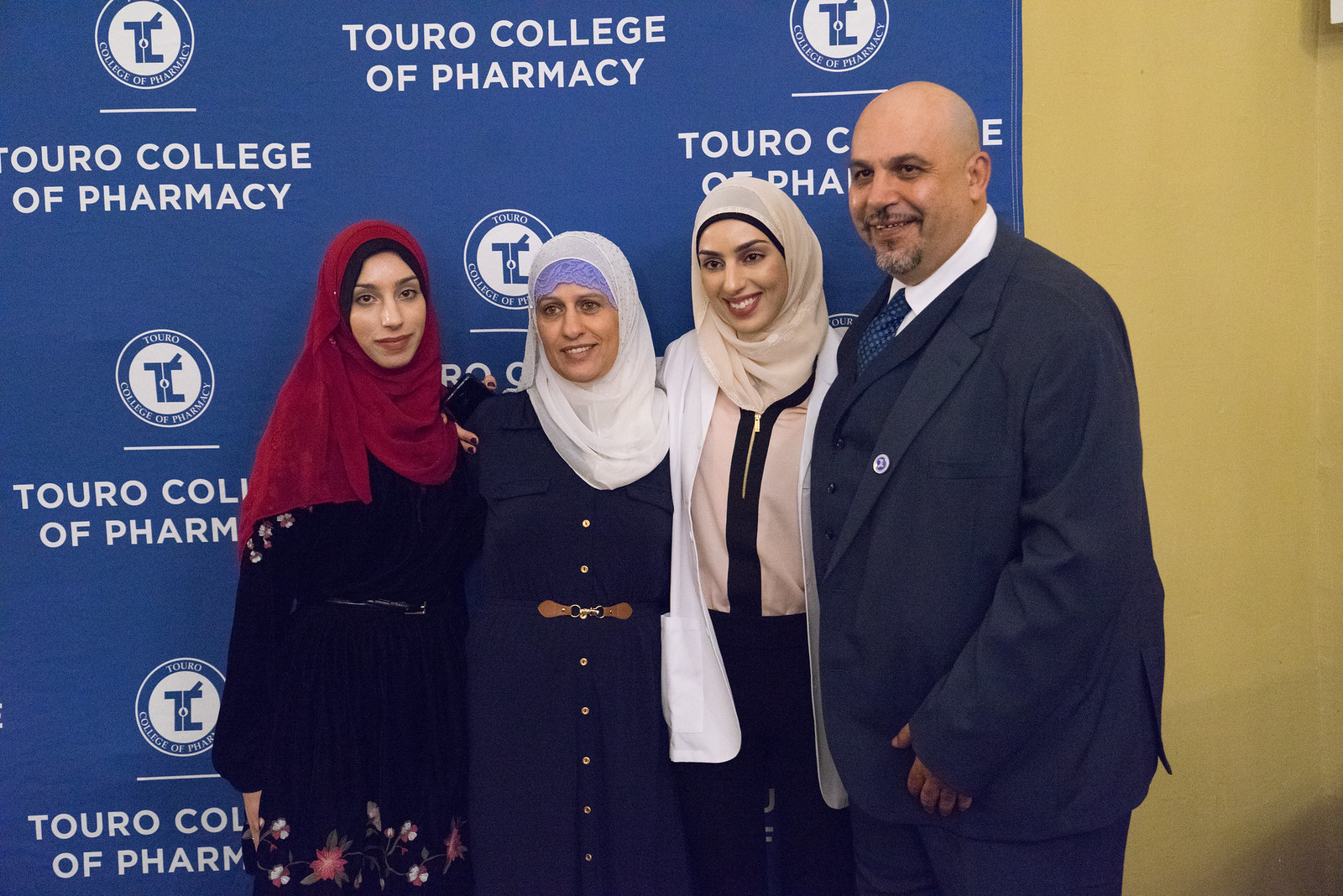The photograph, taken in a room, shows four individuals standing shoulder to shoulder, slightly facing left, and embracing each other. From left to right, the first person is a woman wearing a red hijab and a black dress adorned with designs at the bottom. Next to her is an older woman in a white hijab paired with a dark blue dress. The third person is a woman in a tan hijab, dressed in a black and beige top with black pants. On the far right stands a tall, bald man with a beard and mustache, dressed in a dark suit with a matching vest, a white collared shirt, and a blue tie with white dots. Behind them is a large blue backdrop, covering most of the wall, that reads "Touro College of Pharmacy" in all caps white font, accompanied by the college's emblem. The right edge of the backdrop leaves part of the beige wall visible. All four individuals are smiling warmly at the camera.